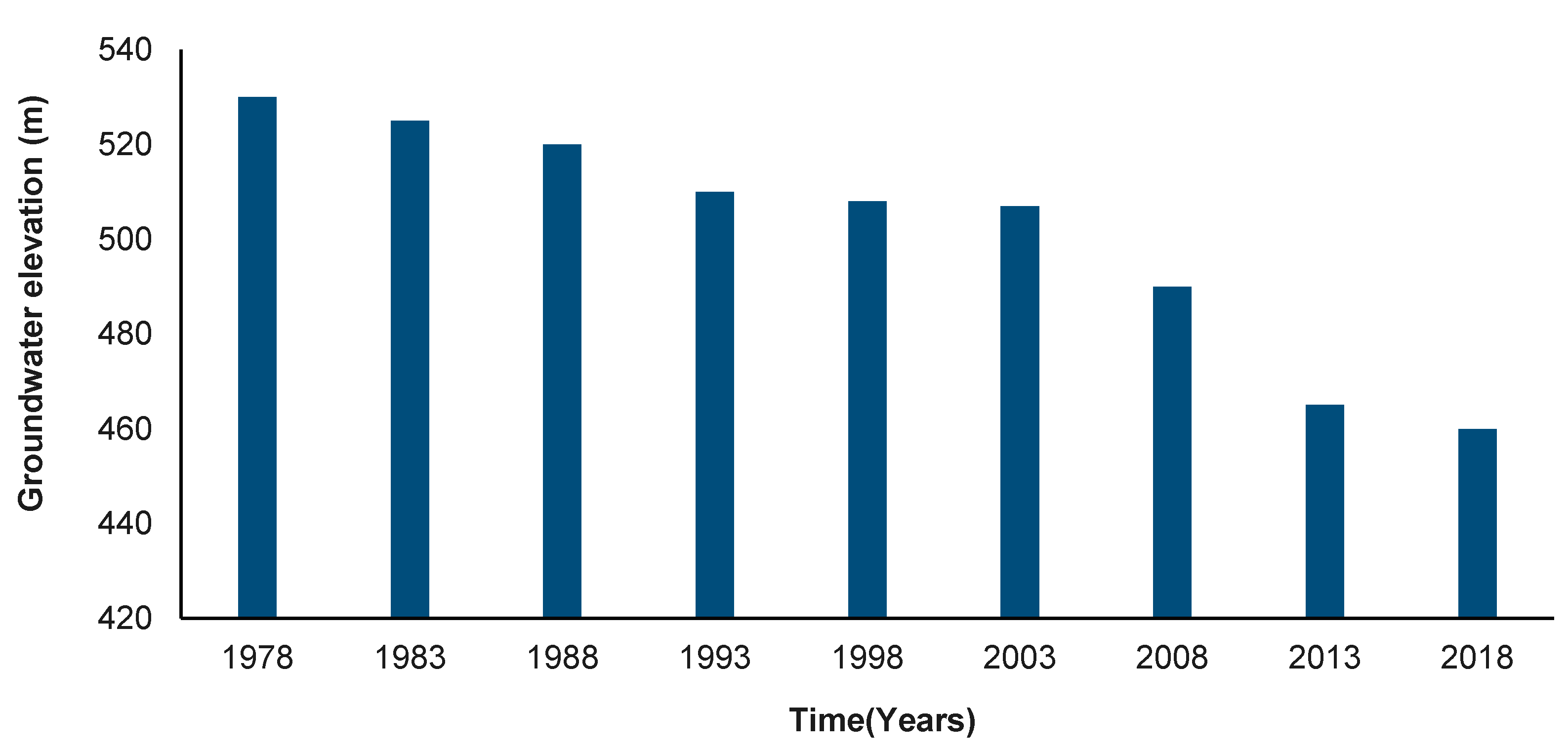This bar chart visually represents groundwater elevation trends over a span of 40 years, from 1978 to 2018. The vertical axis, labeled "Groundwater Elevation (meters)," ranges from 420 meters to 540 meters, while the horizontal axis, labeled "Time (years)," marks the progression of years. The data reveals a clear downward trajectory in groundwater levels over the indicated period. In 1978, the groundwater elevation is at its peak, approximately 530 meters. By 2018, the elevation has significantly decreased, registering at less than or equal to about 460 meters. This decline highlights a substantial reduction in groundwater levels over the four-decade span.